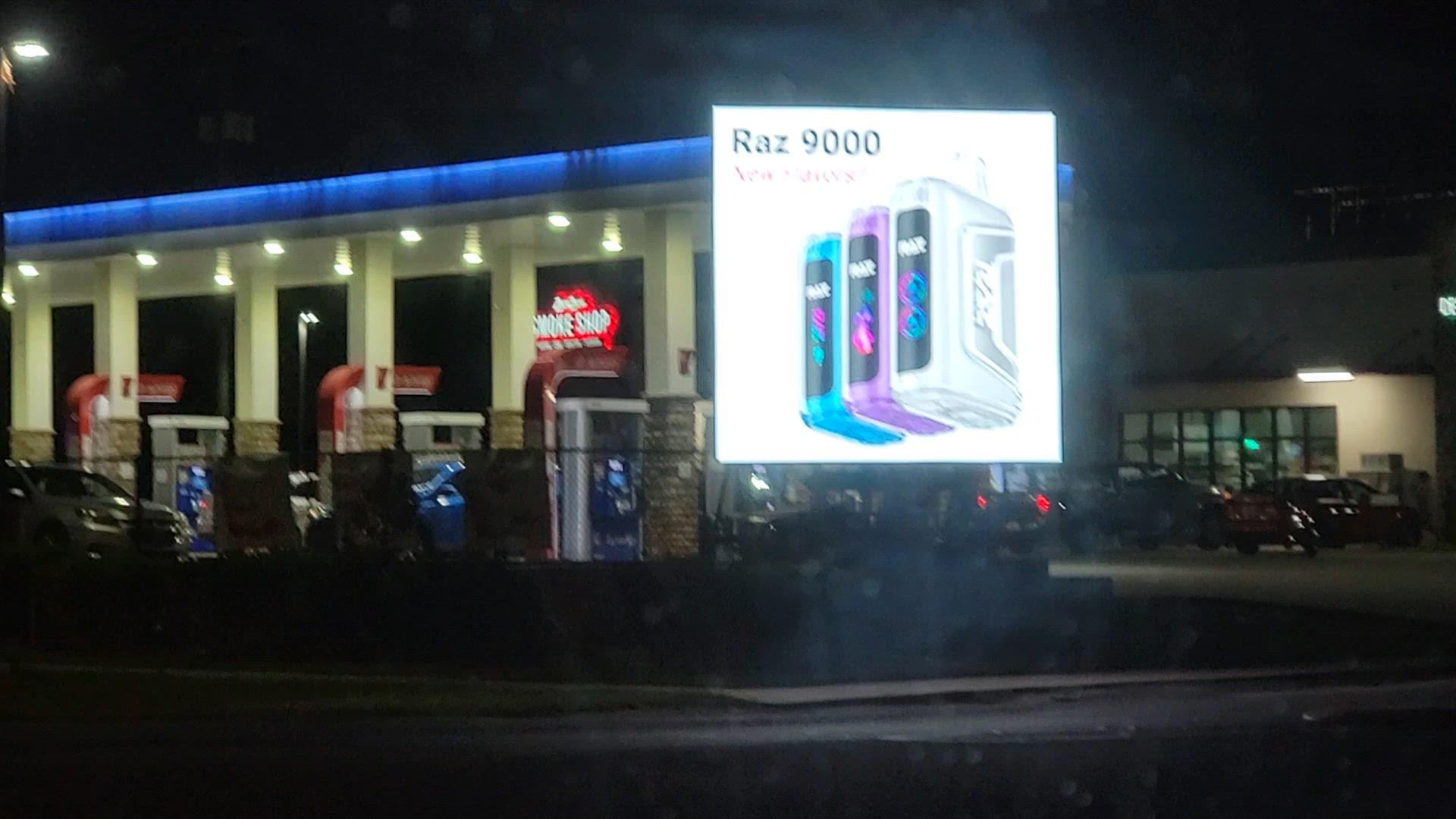The photograph, taken outdoors at night, captures a gas station bathed in the quiet ambience of the evening. The enclosure housing the gas pumps is illuminated by a striking blue neon cylinder that traces its edges, creating an eerie yet beautiful glow against the dark backdrop. Six vertical pillars, painted white, support the structure; their lower halves clad in a variegated brown brick-like material that adds a touch of earthy contrast to the scene. The gas pumps, made of chromed metal and fitted with blue fixtures, gleam under the fluorescent lights. Each pump is adorned with a distinctive curved metal piece that rises gracefully from the bottom edge, arching over the top. 

Embedded within this night-time panorama is an inset featuring the title "RAS 9000" in a white box, highlighting a trio of rectangular devices. Positioned side by side in a neat row, each device is a different color—one blue, one purple, and one white—their right edges perfectly aligned to create a unified display, subtly integrated into the overall composition of the photograph.